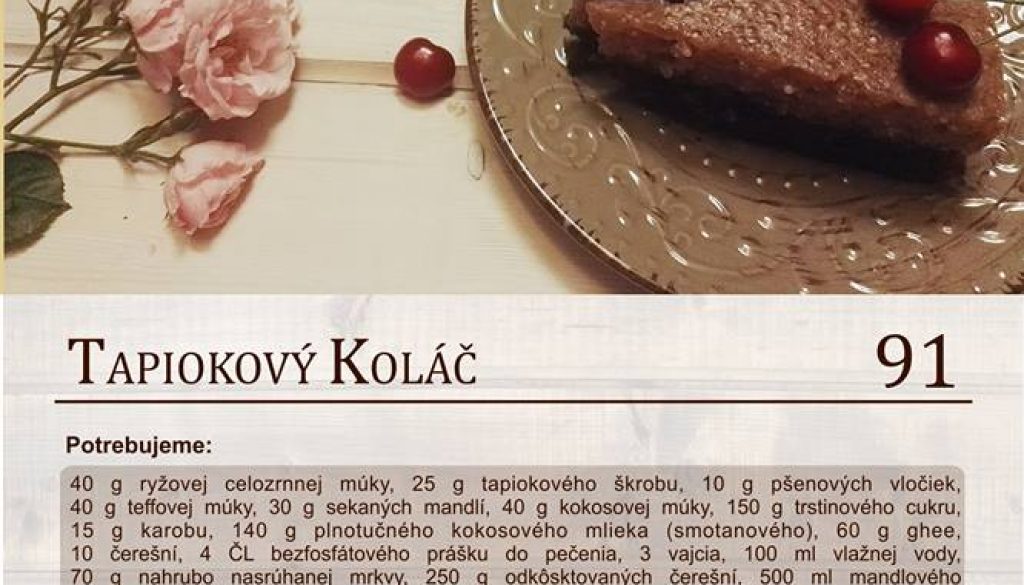The image features a detailed screenshot from a cookbook, predominantly showcasing a recipe in a non-English language, likely an Eastern European one such as Polish. In the top half, there's a vivid image of a dessert, which appears to be a brown slice of cake or flan topped with several cherries. One cherry has notably fallen off the plate onto the table. The cake sits elegantly on a metallic plate adorned with floral designs. To the left, two pink roses with green stems add a touch of natural beauty to the scene. The bottom half of the image contains a white box filled with lines of black text. The main text includes the title "TAPIOKOVY KOLAC 91" followed by a list of ingredients or nutritional information. The colors in the image are mostly muted, with pinks from the roses, browns from the cake, and reds from the cherries, set against off-white and tan backgrounds. This carefully arranged image is primed to guide readers through creating the dessert, indicating its placement in a comprehensive cookbook.